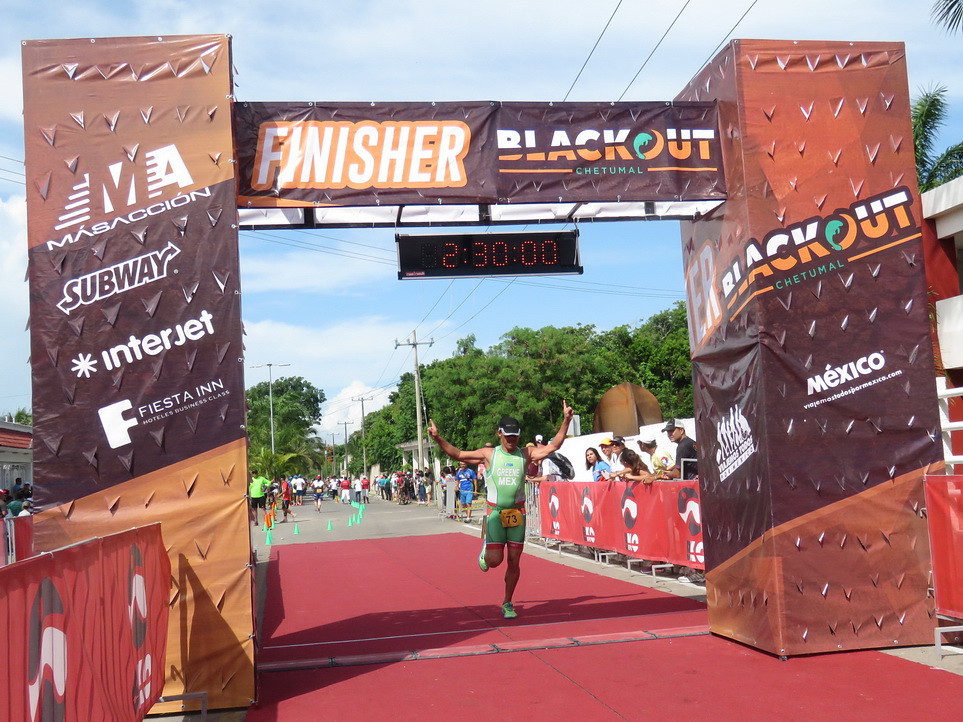In this vivid photograph, a man triumphantly crosses the finish line of a race event in Chutamal, Mexico. His arms raised in a victory gesture, he proudly wears a green sleeveless tank top and matching shorts. His attire is complete with a light green color that extends to his shoes. Clearly visible on his outfit is the entry number 73. The finish line is marked by a red carpeted area and is framed by two towering pillars adorned with logos of various sponsors, including Subway, Interjet, Fiesta Inn, and the event’s primary sponsor, Blackout. Above him, a digital timer prominently displays his impressive finishing time of two hours, 30 minutes, and zero seconds. The top of the structure features a sign that reads “Finisher” against an orange background. Lining the road, enthusiastic spectators are kept back by low steel barriers, as they cheer on the runners against a backdrop of blue skies, fluffy white clouds, trees, and power lines. Additional runners are visible further back, still pushing towards the end of their race.